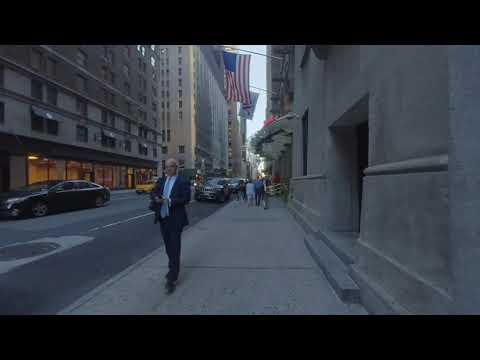The horizontally rectangular image captures a lively city street scene during the day, with dominant hues of gray and teal. The foreground features a bald man wearing glasses, dressed in a dark blue suit with a light blue shirt and tie, walking towards the camera on a wide, light gray sidewalk. To his right is a grayish stone building with a large, curved awning extending towards the sidewalk and displaying an American flag hanging from a pole. Another flag with indistinct initials can be seen further along the building. Behind the man, several people in varying shades of light and dark clothing walk in the opposite direction. The street itself, a dark gray two or three-lane road marked by white lines, is lined with parked cars, including a distinct yellow taxi cab. Across the street, tall, multi-level buildings with numerous windows contribute to the bustling urban atmosphere.